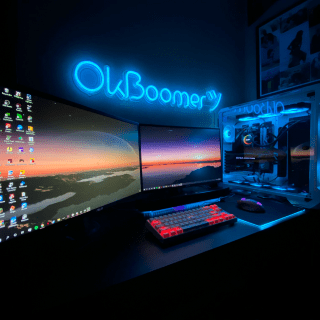The image features a black surface, likely a counter or desktop, extending from the bottom left to the top right. Positioned on this black counter are two monitors, with a large rectangular monitor on the left and another monitor directly beside it. On the far right of the setup, there's an object encased in glass, the details of which are unclear. Above these monitors, a bluish neon sign hangs on the wall, displaying the phrase "OK Boomer" with a small symbol next to it. In front of the monitors, placed on the black surface, is a keyboard featuring a mix of red and black keys; red keys are particularly located on the left, bottom left, bottom right, and a few on the right, while the remainder of the keys are black. To the right of the keyboard lies a mouse, positioned on a mouse pad. The overall scene is cast in a bluish light, contributing to the ambiance of the setup.